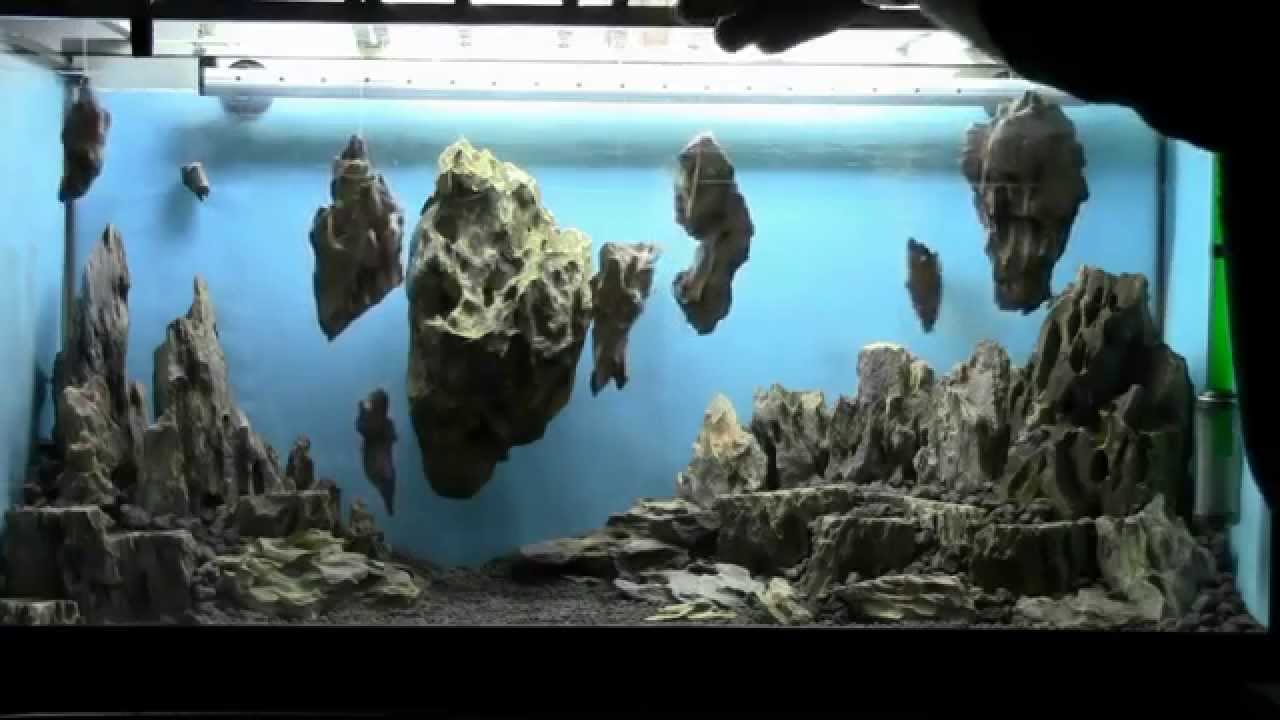The image depicts a moderately-sized indoor aquarium featuring a captivating display of intricately shaped rocks. These rocks, resembling underwater caves and mountains, have a greenish moss-like appearance with grooves and holes that add to their texture. The clear, pale blue water enhances the view, showcasing some rocks anchored to the aquarium floor while others appear to be floating, particularly in the center and towards the right. The floating rocks are mostly dark with lighter elements scattered throughout. The background of the aquarium is a baby blue color that contrasts with the black shadowed figure of a man's arm and fingers grasping the lid in the right corner. Additionally, a green tube is visible in the right part of the image, and there is a white beam and ceiling structure at the top, completing the scene.